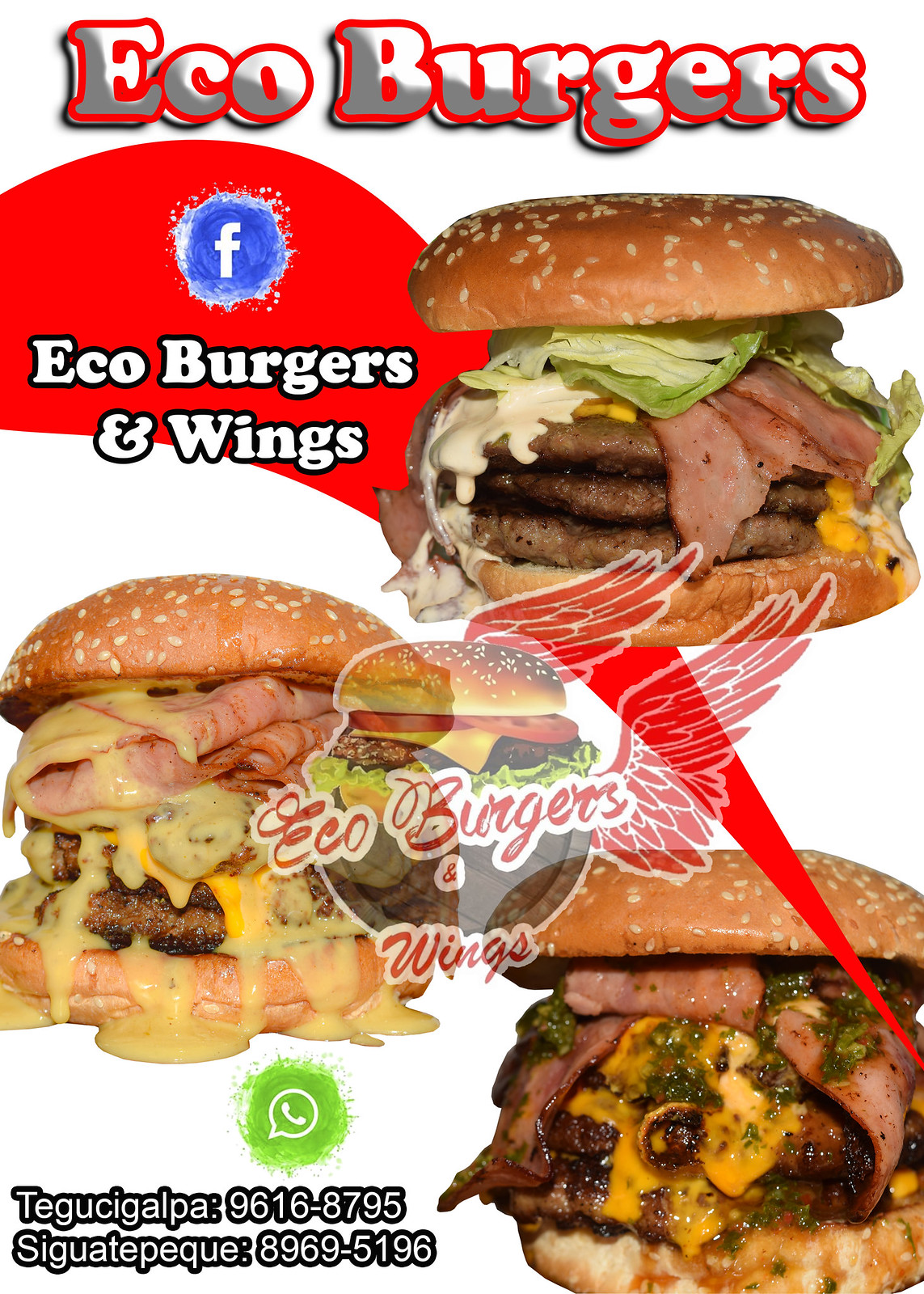This advertisement flyer for Eco Burgers and Wings showcases three massive, triple-decker burgers loaded with various meats and toppings. The top of the flyer features the name "Eco Burgers" in white and gray letters outlined in red, set against a white background with a red swoosh extending from the upper left to the lower right. Underneath the swoosh, the text reads "Eco Burgers and Wings" in white with a black border. A Facebook logo is prominently displayed above this text, indicating the establishment's social media presence.

The flyer is dominated by illustrations of three enormous and enticing burgers. The first burger appears with three patties, lettuce, and ham. The second burger features turkey layered over two patties topped with oozing melted cheese. The third burger is adorned with bacon alongside its three patties, also dripping with melted cheese and sauce. These burgers look mouthwateringly delicious but also notably messy to eat.

In the center of the flyer, there is a semi-transparent image of another burger with wings, suggesting it is flying across the picture, emphasizing the dynamic and playful branding of Eco Burgers and Wings. At the bottom is a green circle containing a telephone symbol, accompanied by two phone numbers: 9616-8795 and 8969-5196, indicating ways to contact the establishment, possibly via WhatsApp. The entire flyer emphasizes the substantial and indulgent nature of the burgers, making them appear highly appealing yet undeniably messy.